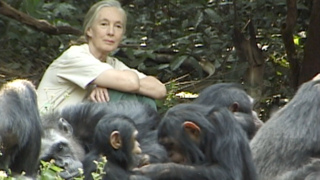In this captivating image, a Caucasian woman with gray hair pulled back, possibly resembling Jane Goodall, is sitting in a densely wooded forest. She is dressed in a white t-shirt and is seated on the ground with her knees pulled up to her chest and her arms crossed over them. The background is rich with tree trunks and foliage, indicating a heavily wooded area. In front of her, a multitude of black monkeys with brownish ears are gathered, creating a sense of intermingling and closeness. Her expression is a mix of alertness, amusement, and pensiveness as she looks directly at the camera. The monkeys vary in age and size, with at least five of them clearly visible in the foreground. Some are sitting upright while others lay sprawled on the ground, contributing to a dynamic and lively scene where the woman and the monkeys share a serene moment in nature.